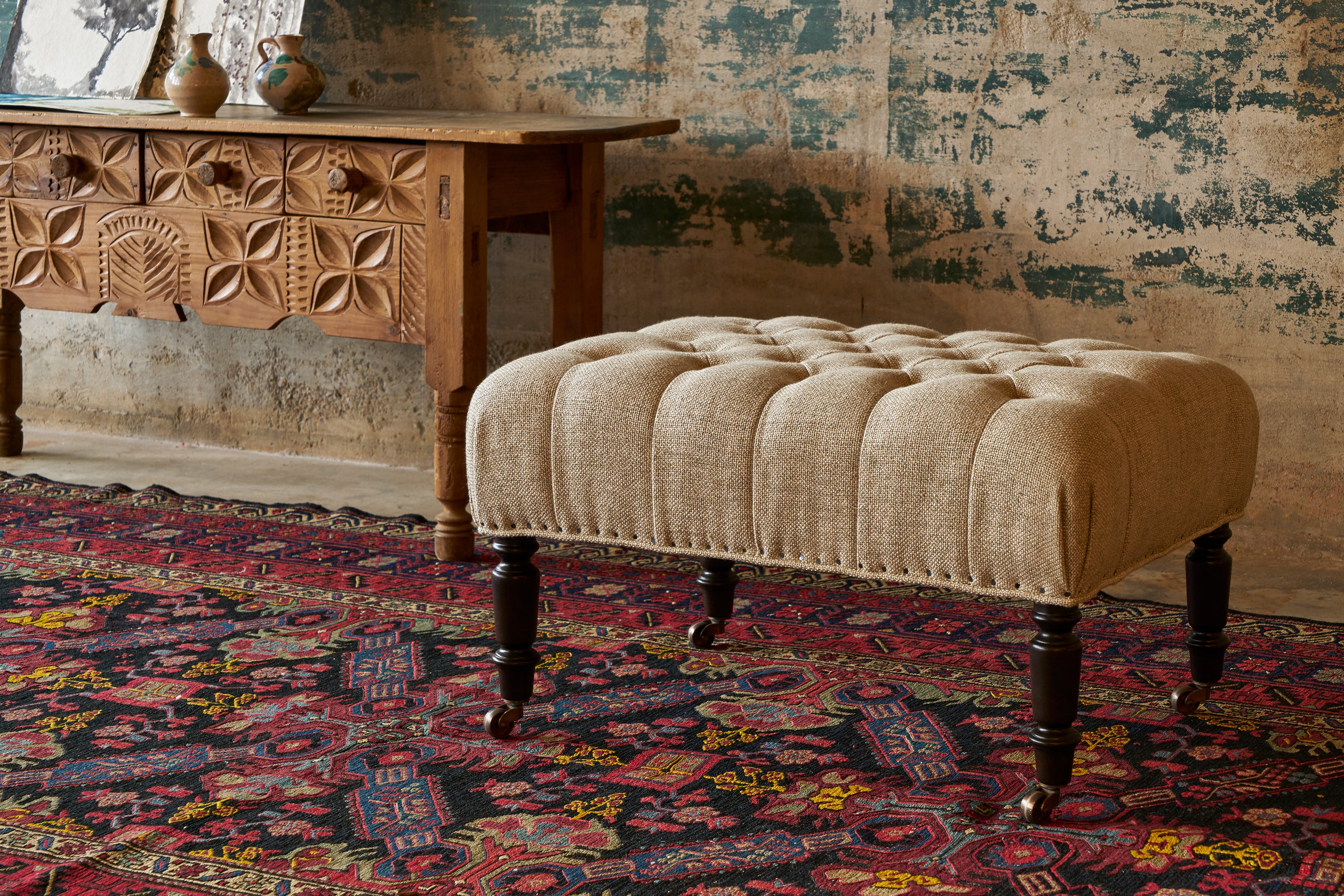The photograph captures a detailed indoor scene featuring a close-up of a tan-colored ottoman with dark brown wooden legs and small wheels, upholstered in a fancy fabric with recessed buttons adding texture to the top. The ottoman rests on an intricately patterned, vibrant oriental carpet with dominant colors of maroon, red, blue, yellow, green, and dark blue. Behind the ottoman stands an ornate, light brown antique table, possibly a drop-leaf style, with carved floral designs on its sides. On top of the table sit two terracotta clay vases and two black and white photographs, one depicting a tree and the other indistinguishable. The backdrop consists of a distressed concrete wall with green and tan hues, possibly featuring a mural that's not fully visible.